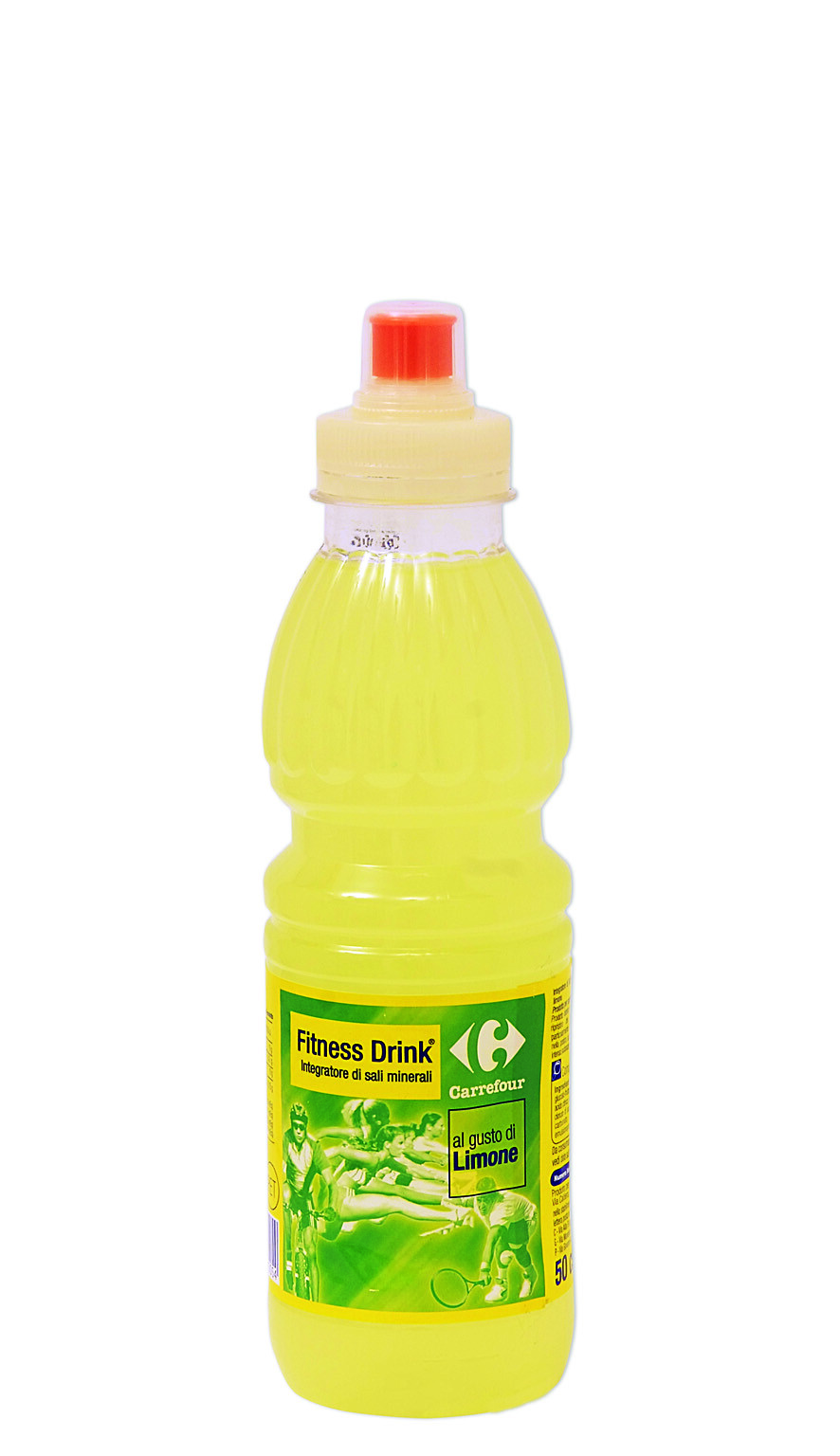This image features a plastic bottle containing a pale yellow fitness drink with minerals, likely lemon-flavored, as indicated by the label reading "Augusto Limone." The drink is bottled in a narrow, clear plastic container, which contains approximately 16 to 20 ounces. The bottle has an orange pull-up spout for easy drinking and a white screw-on cap that helps keep the spout clean when not in use. The label is predominantly green and white, with some gold accents, and it features various action images. These include illustrations of people engaging in activities such as tennis, swimming, bike riding, weight lifting, racing, and possibly gymnastics. The label also prominently displays the Carrefour logo, indicating the brand. The background of the image is entirely white, without any additional objects or borders.